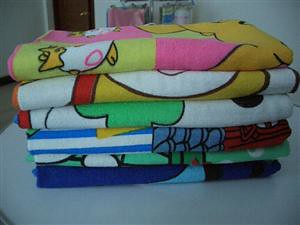The image is a small, low-resolution photo taken in landscape format, featuring a neatly stacked pile of six vibrant fabrics, likely beach towels due to their intricate designs. These towels, folded uniformly and placed on a white surface, display a range of colorful patterns, though the exact designs are somewhat indistinct. The top towel features a mix of orange, pink, yellow, and white hues, possibly evoking a playful image like Winnie the Pooh. The second towel shows a combination of white, red, and tan, which might depict a clown face. The third towel includes patches of white, green, and black, while the fourth sports blue and white stripes with some yellow. The fifth towel is blue with black circles and red accents, and the bottom towel is dark blue interspersed with lighter blue tones. The photo is set in a room with white walls; in the background, a door is visible on the left, accompanied by hints of pink and blue items along the wall, likely cleaning products or toiletries, adding context to the domestic setting.